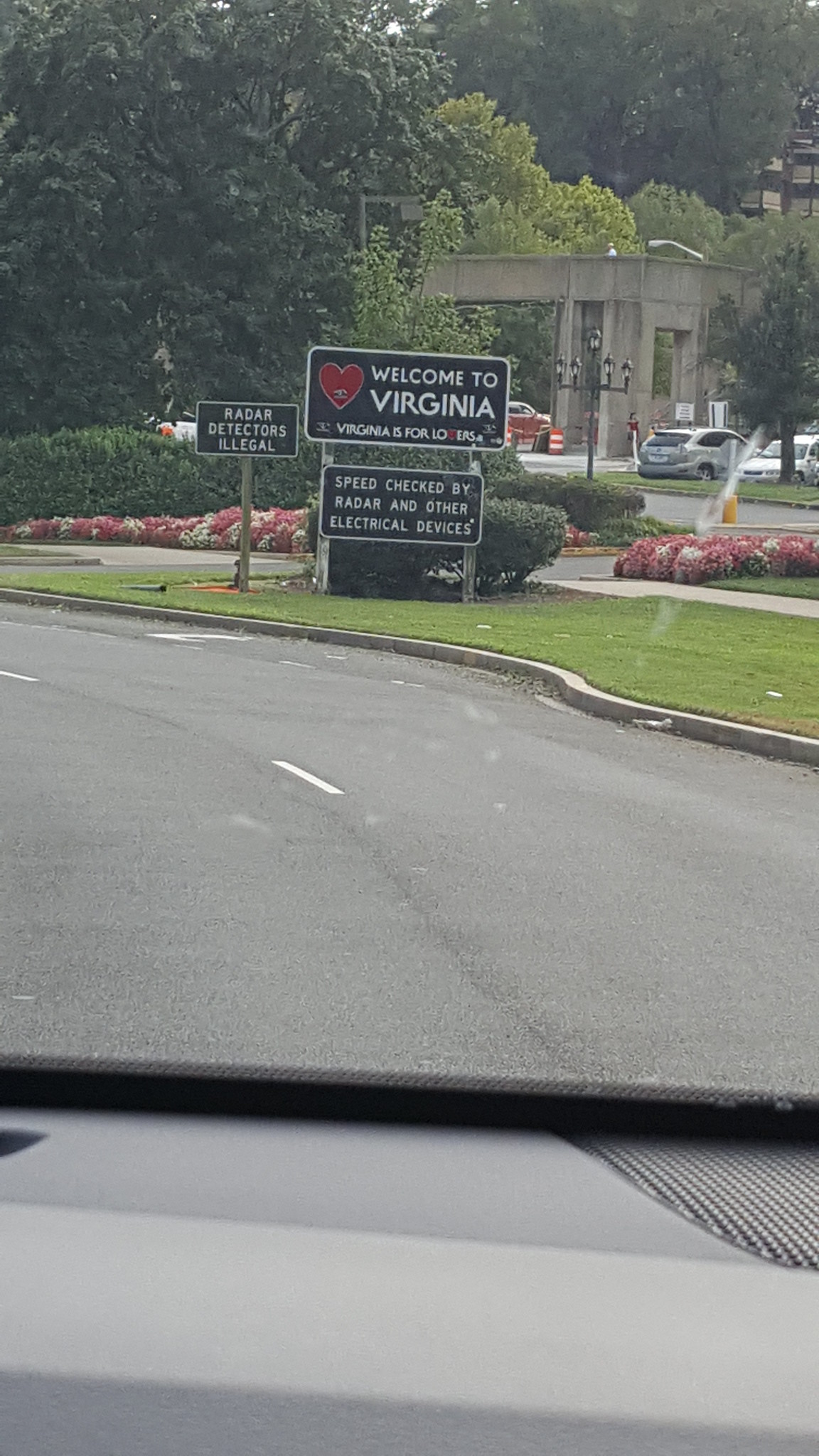This photograph captures a view through the windshield of a car, with a small portion of the dark grey and black dashboard visible at the bottom. The scene extends onto a paved road marked with white lane dividers. To the right, a grassy median is adorned with a delightful array of pink and white flowers. Atop this median, several street signs are prominently displayed. 

The uppermost sign is a rectangular, rounded-edged sign that warmly welcomes visitors, stating, "Welcome to Virginia," accompanied by the slogan "Virginia is for lovers" and accentuated by a red heart. Beneath it, another sign warns that the "Speed checked by radar and other electrical devices." A standalone post to the left holds a sign declaring, "Radar detectors illegal."

In the background, a parking lot and a cluster of trees can be seen, contributing to the composition of this vibrant roadside snapshot.